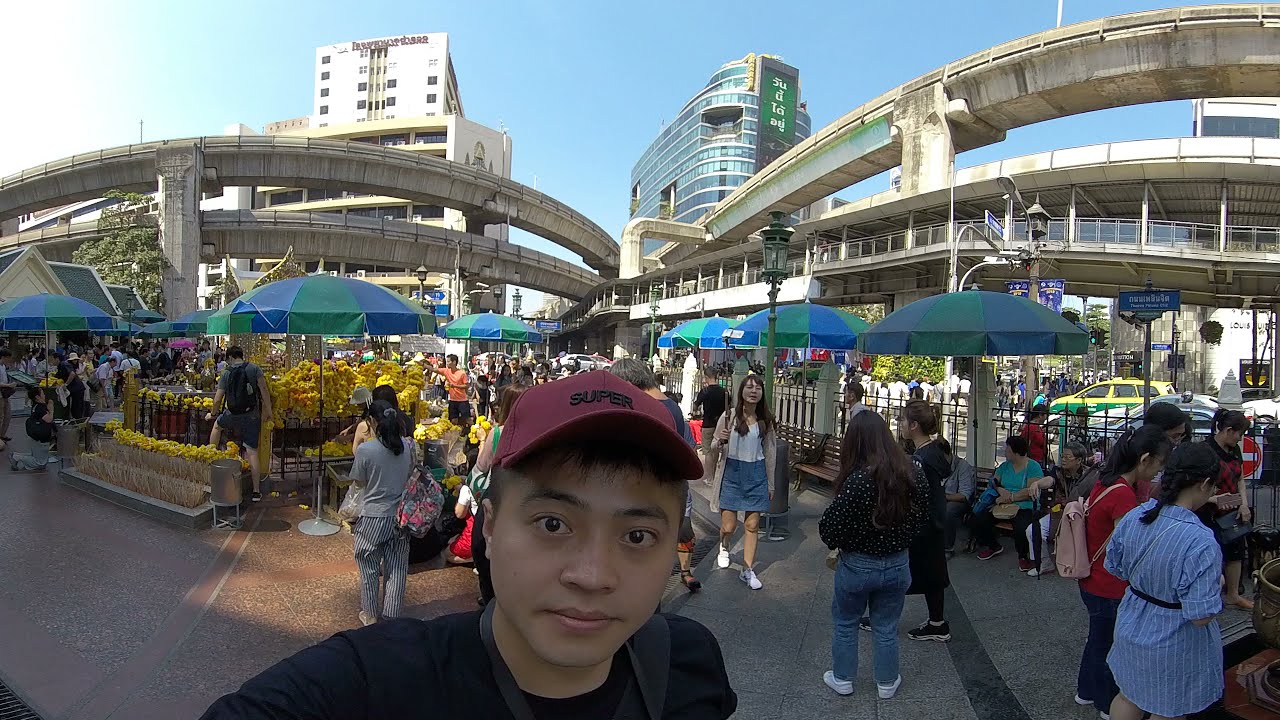In this bustling and vibrant outdoor scene, we see a young man taking a selfie in the foreground. He sports a maroon cap with the word "super" in black lettering, has dark hair and eyes, and wears a neutral expression as he looks directly at the camera. The image is full of life with numerous people milling about, indicating a busy, possibly touristy area in an Asian city, likely Japan or China, as suggested by the surrounding signs in Asian characters.

The setting is a hard-tiled surface, and towards the bottom of the image, a gate prevents people from entering the road directly. The center is crowded with people walking and chatting, some sheltered under pop-up umbrellas in blue and green, creating shaded areas. Off to the left, there are market stalls, possibly selling yellow flowers or food.

In the background, elevated trains or narrow highways criss-cross above the scene, leading up to the taller multi-story buildings typical of a dense urban environment. The leftmost building appears to be clad in stone or plaster, while a blue, glass-covered structure stands to the right. Above it all, the sky is clear and blue, hinting at a bright, sunny day.